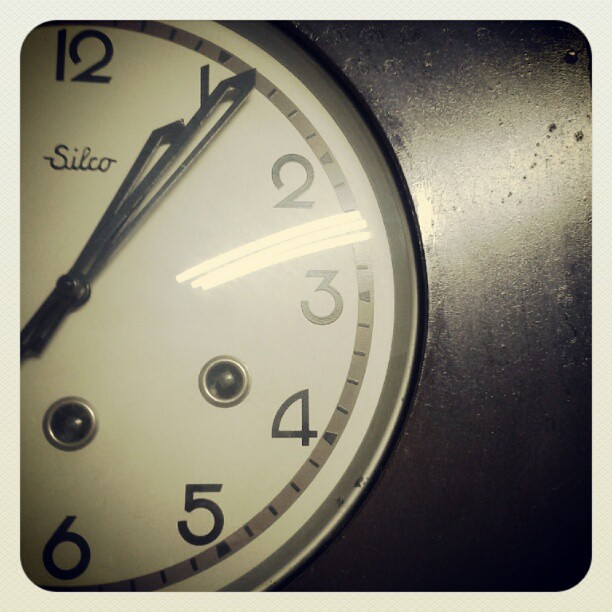The image showcases the upper half of a classic school wall clock, characterized by its black paneling and a translucent glass or plastic cover. The clock face is adorned with large black numerals arranged in a clockwise direction, displaying the numbers 12, 1, 2, 3, 4, 5, and 6. Prominently featured are the black hour and minute hands, both tapering to precise points, indicating the time as approximately 1:06. Additionally, there are two small, silver areas on the clock’s face, which may function as indicators for lighting up or signaling the time for recess or dismissal, possibly serving as bell chimes. The overall design and features are typical of clocks found in educational settings.